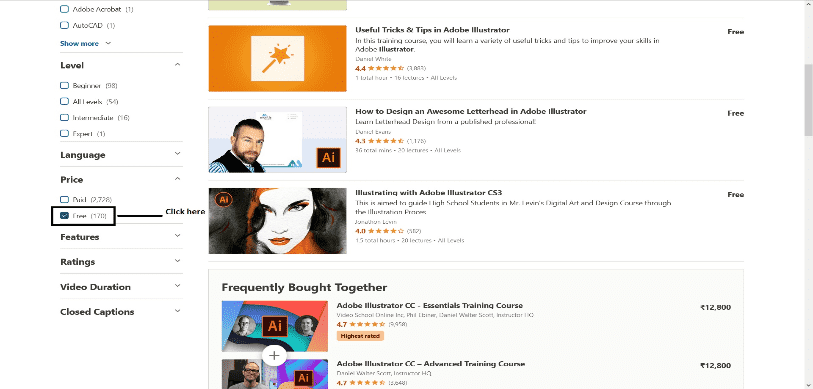The interface displays a list of selectable criteria on the left-hand side, including level, language, price, features, rating, video duration, and the availability of closed captions. On the right side, it features thumbnails of various courses with descriptions and prices aligned to their right.

From the top, the first course is titled "Useful Tricks and Tips in Adobe Illustrator." The description reads, "In this training course, you'll learn a variety of useful tricks and tips to improve your skills in Adobe Illustrator." This course has a rating of 4.4 stars and is available for free.

Following that is "How to Design an Awesome Letterhead in Adobe Illustrator," rated at 4.1 stars and available for free.

Next is "Illustrate with Adobe Illustrator CS or CS3". Some text is unreadable here, but below it mentions a frequently bought-together option: "Adobe Illustrator CC Essential Training Course," priced at 12,800, holding a rating of 4.7 stars.